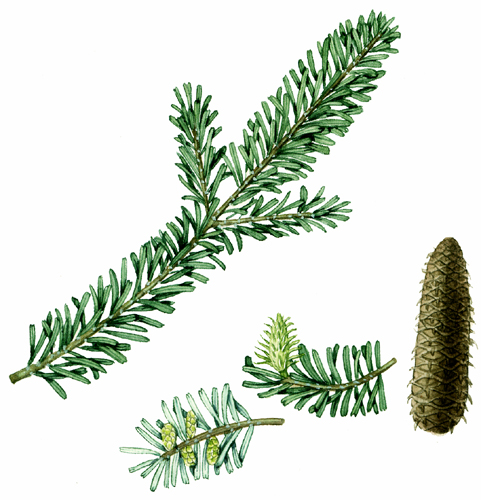This detailed, textbook-style diagram features different stages of pine cone development on a pine tree, meticulously rendered in a realistic illustration. The main focus is on various growths of pine cones and branches, all set against a simple white background with no extra contextual elements. 

Starting from the left side of the image, a small branch with light-colored, almost white leaves, carries multiple blooming pine cones. Just to the right, a smaller branch with leaves showcases a single young pine cone attached to it. Further to the right, there's a standard, mature pine cone depicted vertically, characterized by its long, slightly brownish-green appearance, similar in shape to an elongated cob. Above these elements, a longer stretch of a branch runs diagonally from the lower left to the upper right corner of the image. This branch has vibrant green leaves extending from it and two smaller branches that diverge from its middle section.

The artwork is a precise and lifelike drawing that effectively mimics the detailed nature of botanical illustrations typically found in educational textbooks.